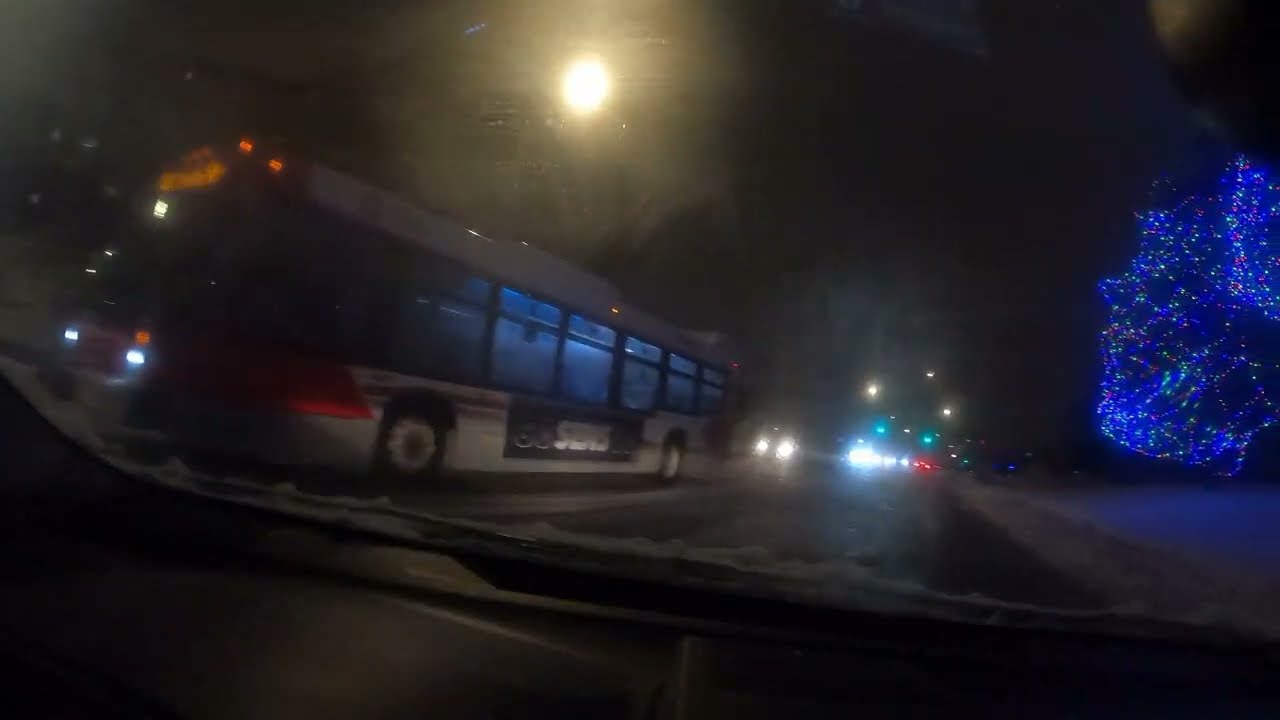The photograph captures a nighttime winter scene from the perspective of a driver looking out the windshield of a car. The windshield is partially covered in snow, with the wipers visible. The car is driving in the right lane of a snow-covered road. On the left side of the road, a white city bus with a black advertisement panel and blue-lit windows is about to pass by, followed by other headlights in the distance. The right side of the image shows a patch of snow and a tree adorned with blue Christmas lights. The upper half of the image is dominated by a black sky, punctuated by a bright street light slightly off-center to the left. In the far distance, there are faint green traffic lights. The overall scene is cold and wintry, with a mixture of artificial lights providing contrast in the dark night.